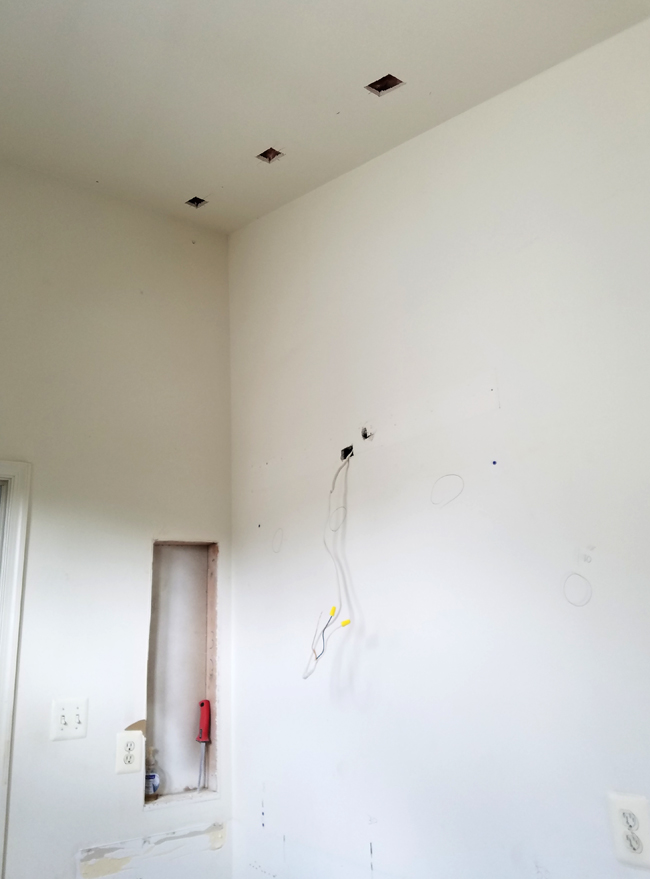The image depicts an interior room with stark, white walls on both the left and right sides as well as the ceiling, creating a clean and sterile ambiance. Dominating the bottom right corner is a standard white electrical outlet featuring two sockets. The top middle section of the ceiling showcases three square holes arranged in a diagonal pattern, descending from the top right to the middle left. Adjacent to them, slightly to the right of the center, is a rectangular hole with a white wire extending out of it. The wire splits into two smaller wires, one blue and one red, each with a small yellow sponge-like attachment at the end. On the far left edge of the image, a white door frame can be partially seen. Positioned to the right of the door frame, in the bottom left corner of the image, are two downward-facing white light switches. Just below these switches lies a screwdriver with a red handle, completing the scene.